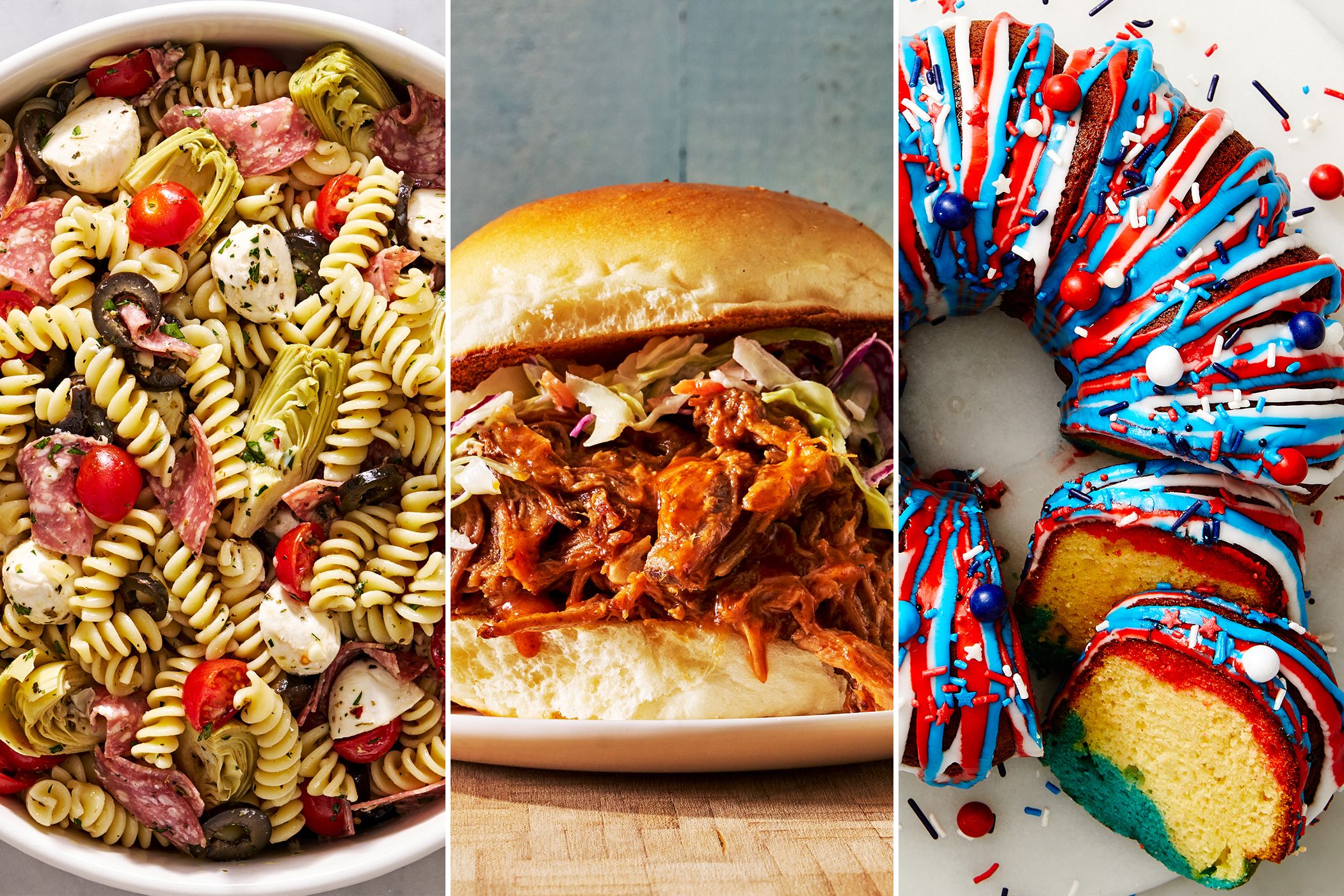This captivating montage features three tantalizing food photographs. On the left, there's a vibrant top-down view of a hearty pasta salad, beautifully arranged in a white bowl. The salad is a colorful medley of spiral rotini noodles, savory slices of salami, juicy cherry tomatoes, briny black olives, and crunchy bits of red cabbage, all enhanced by chunks of creamy white cheese. The center photograph showcases a sumptuous pulled pork burger, presented side-on atop a white plate on a rustic wooden table. This generously filled burger boasts tender, saucy pulled pork sandwiched between a fluffy, perfectly toasted bun and is topped with a crisp coleslaw featuring red cabbage. On the right, a festive Bundt cake steals the spotlight with its patriotic red, white, and blue theme. Captured from above, this cake is adorned with vibrant stripes of icing and sprinkled with matching colored buttons. Two moist yellow cake slices have been neatly plated on their sides, ready to be served.